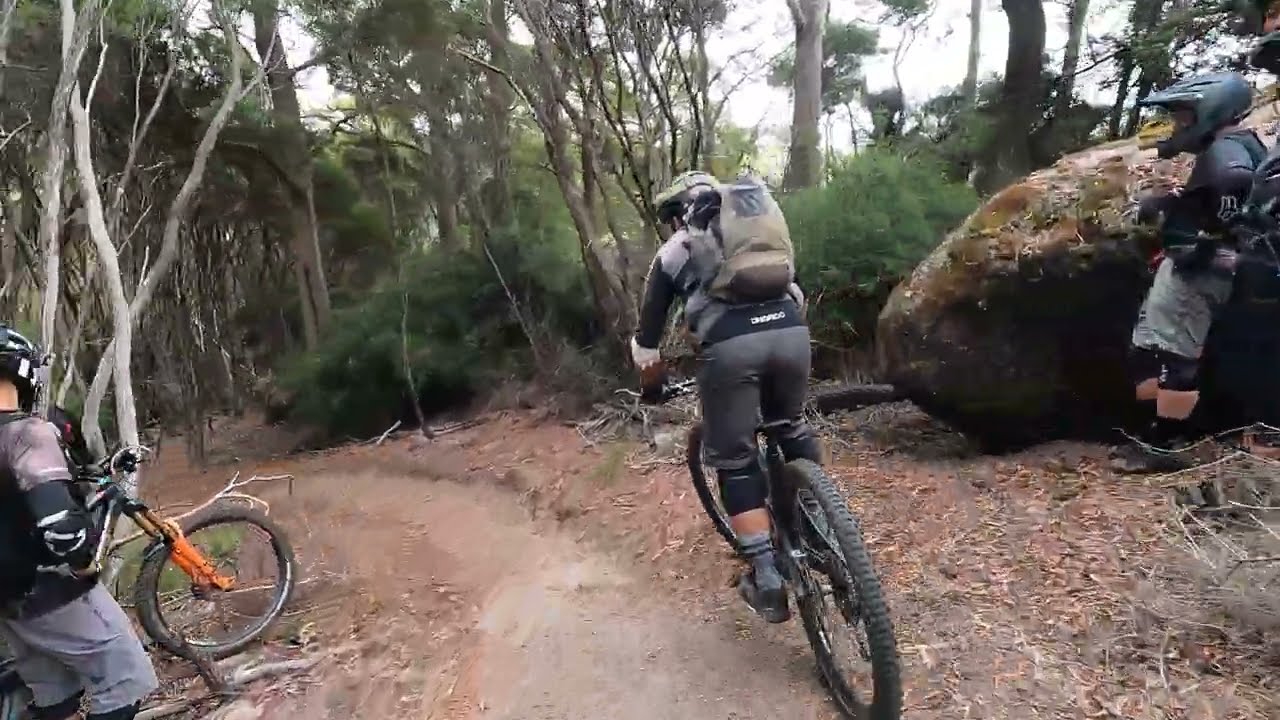A full-color, slightly out-of-focus photograph taken outdoors during the daytime captures a horizontally rectangular scene of a dirt bike trail winding through a dense wooded area. The trail curves sharply to the left and descends, surrounded by tall trees, dead leaves, and debris scattered on the ground. Prominently positioned on the right side is a massive boulder against which one of the three helmeted mountain bikers is leaning. Each biker is wearing distinctively colored top and bottom gear along with gloves and backpacks. In the lower left corner stands another biker beside their dirt bike, while a third biker rides along the trail in the center of the image. The overall scene is bathed in daylight, highlighting the natural and rugged terrain of the trail.